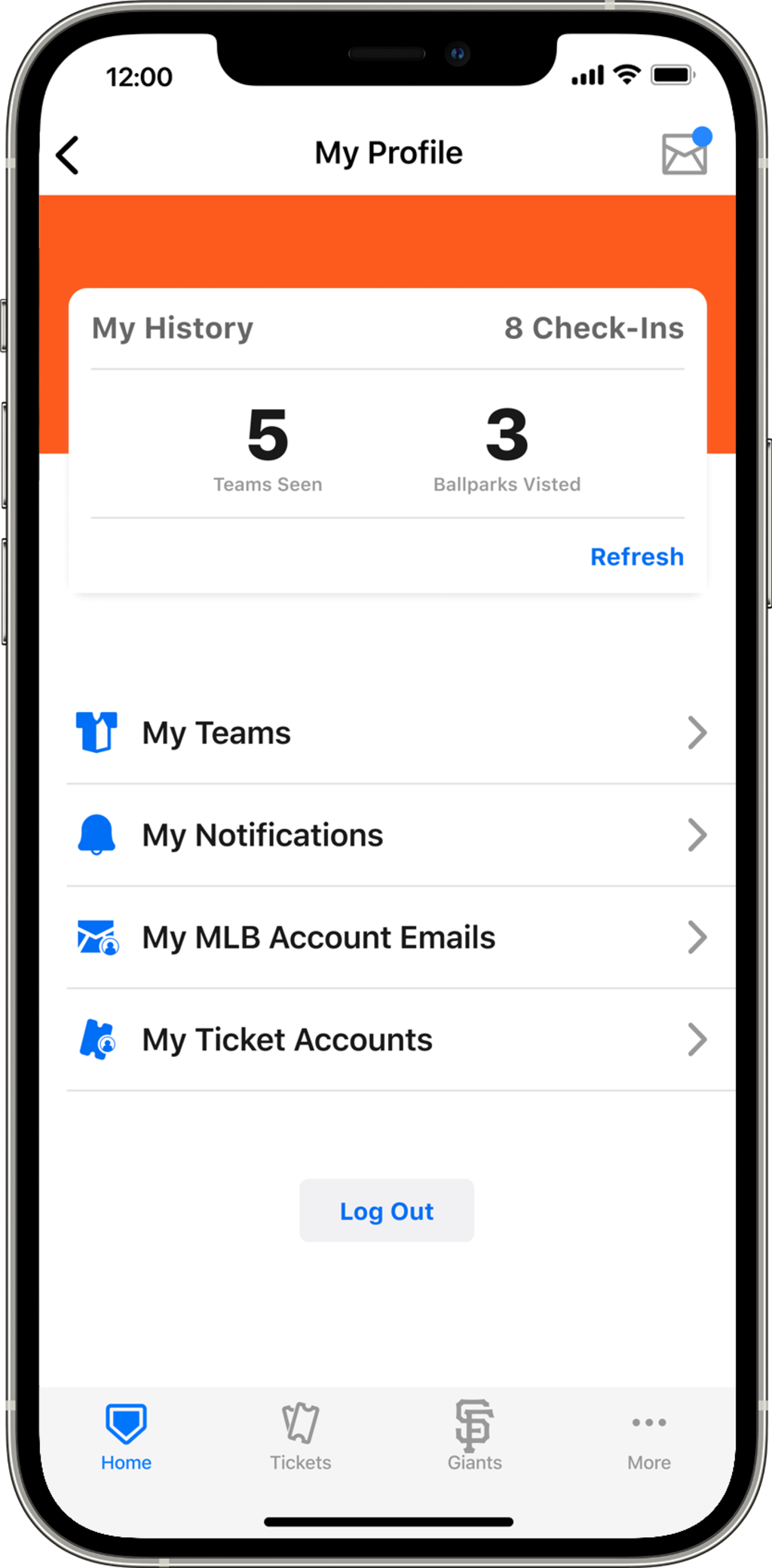A detailed view of someone's cell phone screen is displayed, showcasing their MLB app profile. The screen prominently features a header labeled "My Profile" followed by various sections including "My History" and "Eight Check-ins." Below this, it states "Five Teams Seen" and "Three Ballparks Visited." A "Refresh" button is visible in the lower right-hand corner of the screen.

Further down, there are icons accompanying different categories: a jersey icon labeled "My Teams," a bell icon labeled "My Notifications," an envelope icon labeled "My MLB Account Emails," and a ticket icon labeled "My Ticket Accounts." At the very bottom of the screen, "Log Out" is displayed in blue text.

Near the bottom navigation bar, an icon resembling a shield or home plate beside the word "Home" is visible, followed by "Tickets" and "Giants" identified by the letters "S" and "F." There is also a "More" tab accompanied by three horizontal dots.

The top of the screen features an orange rectangle background with "My History" and "Eight Check-ins" emphasized. The status bar shows it is 12 o'clock, with almost a full battery charge visible.